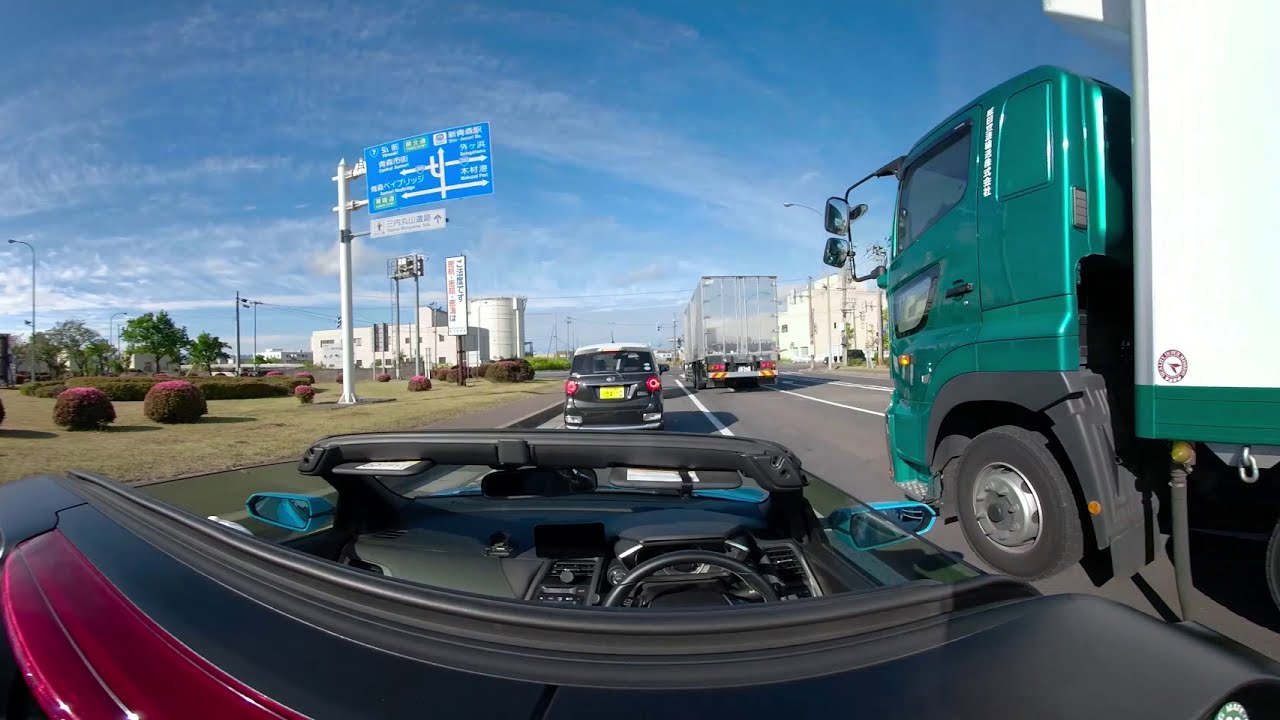The rectangular photograph captures a clear, sunny day on a busy highway, taken from behind a convertible vehicle with its top down, but no occupants inside. The black convertible is driving in the left-hand lane, with visible red taillights. To the right of the convertible is a large green semi-truck with a white trailer, and in front of this truck is another semi-truck with a silver trailer. Directly ahead of the convertible in the same lane is a black minivan or SUV with a yellow license plate. The upper left side of the image features an overhanging blue highway sign with white text, likely in Chinese, suggesting the location is in China. The background reveals tall buildings on either side and a bright blue sky interwoven with thin, white fluffy clouds. Grass and bushes are also visible to the left of the highway.